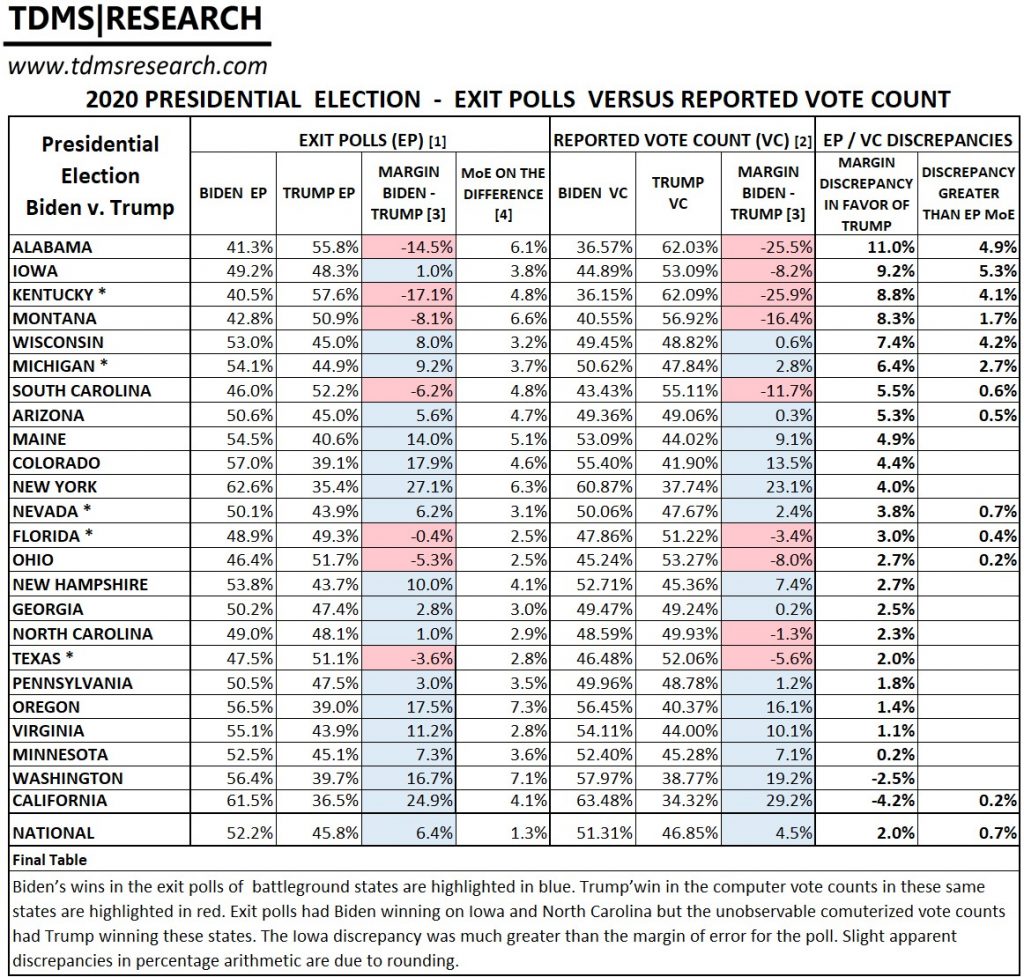Here is a cleaned-up and detailed caption for the image:

---

This screenshot is taken from the TDMS Research website, found at www.tdmsresearch.com. The image focuses on the 2020 Presidential Election, comparing two exit polls with the reported vote count. Central to the image is a detailed table presenting election results for President Joe Biden versus President Donald Trump. The table includes several columns:

1. **States** listed where the elections were held.
2. **Overall win rates** indicating the percentage of votes each candidate received in each state.
3. **Exit poll percentages** for both candidates.
4. **Difference percentages** between the exit polls and the official vote counts.

Additionally, the reported vote counts for both Biden and Trump are shown, alongside the margin of loss or victory for each candidate in each state. The spreadsheet is color-coded, using blue to signify Democratic wins and red for Republican victories, clearly delineating the voting outcomes by party.

---